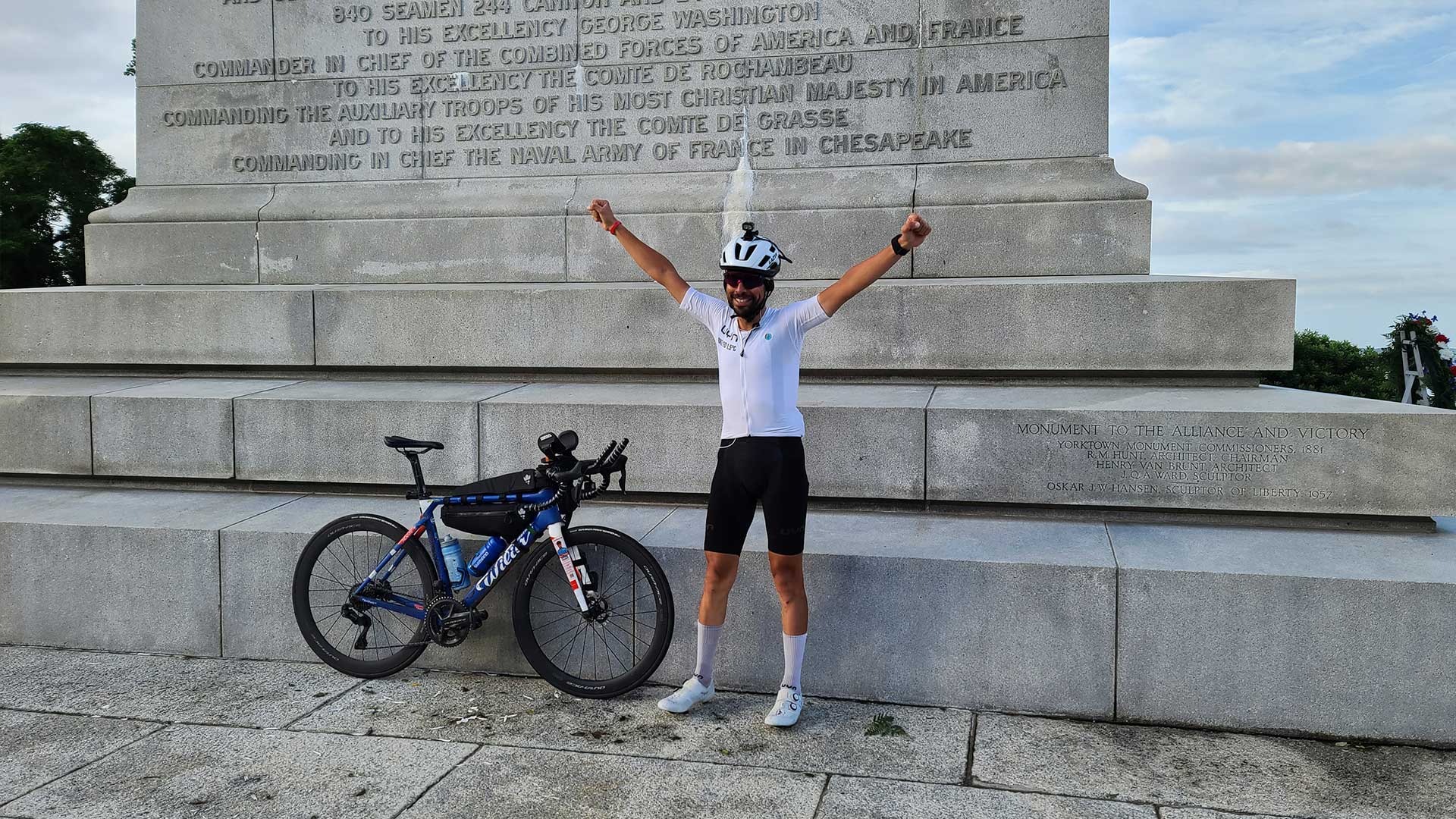The photograph captures a young man, seemingly in his late 20s, celebrating triumphantly in front of a grand, historical monument dedicated to George Washington and his troops. The man, dressed in bicycling attire with a tight white shirt, black shorts extending to his knees, light purple socks reaching his shins, white athletic shoes, and a distinctive white helmet adorned with a GoPro, is striking a victorious pose with his arms raised in a V formation. His bike, sporting a blue frame with dark blue trim and white lettering, leans against the monument’s base. The monument itself is an aged, gray structure with three ascending steps and extensive engraved text, including "Monument to the Alliance and Victory." The background reveals a partly cloudy blue sky with trees framing the scene—a large tree to the left and a distant cluster to the right—all set against a stone slab ground marked with black splotches.